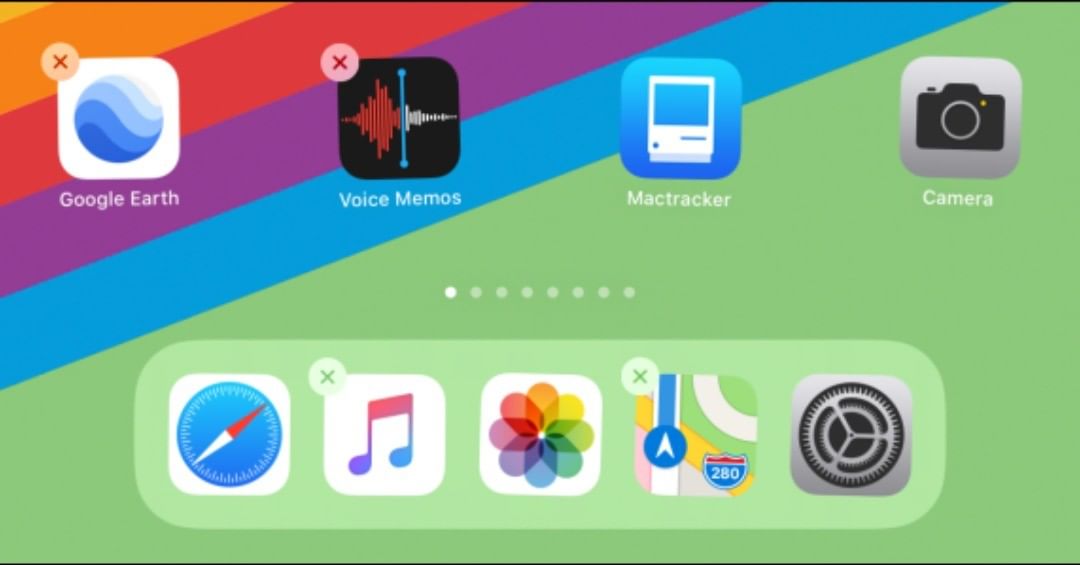This image is a high-resolution screenshot taken on a mobile device, likely an iPad, in landscape orientation. The background is a striking diagonal rainbow gradient, starting with a vibrant orange band in the top left corner, transitioning through dark red, purple, and blue. These colorful bands occupy nearly half the image, stopping just short of the midway point. The remaining background is filled with a muted olive green color.

In the top right corner of the screen, four app icons are arranged from left to right: Google Earth, Voice Memos, Mac Tracker, and the Camera app. The Google Earth icon features a multi-shaded blue globe on a white square background. The Voice Memos icon is a black square adorned with a red and white waveform graphic. The Mac Tracker app icon is blue with an illustration of an old iMac computer. Lastly, the Camera app icon is a gray square with a black camera symbol.

At the bottom of the screen is the Favorites dock, displaying another set of four icons: Safari (a blue compass on a white background), iTunes (a multicolored musical note on a white background), Photos (a multi-colored flower), Maps (a map illustration), and the Settings app (a series of grey gears).